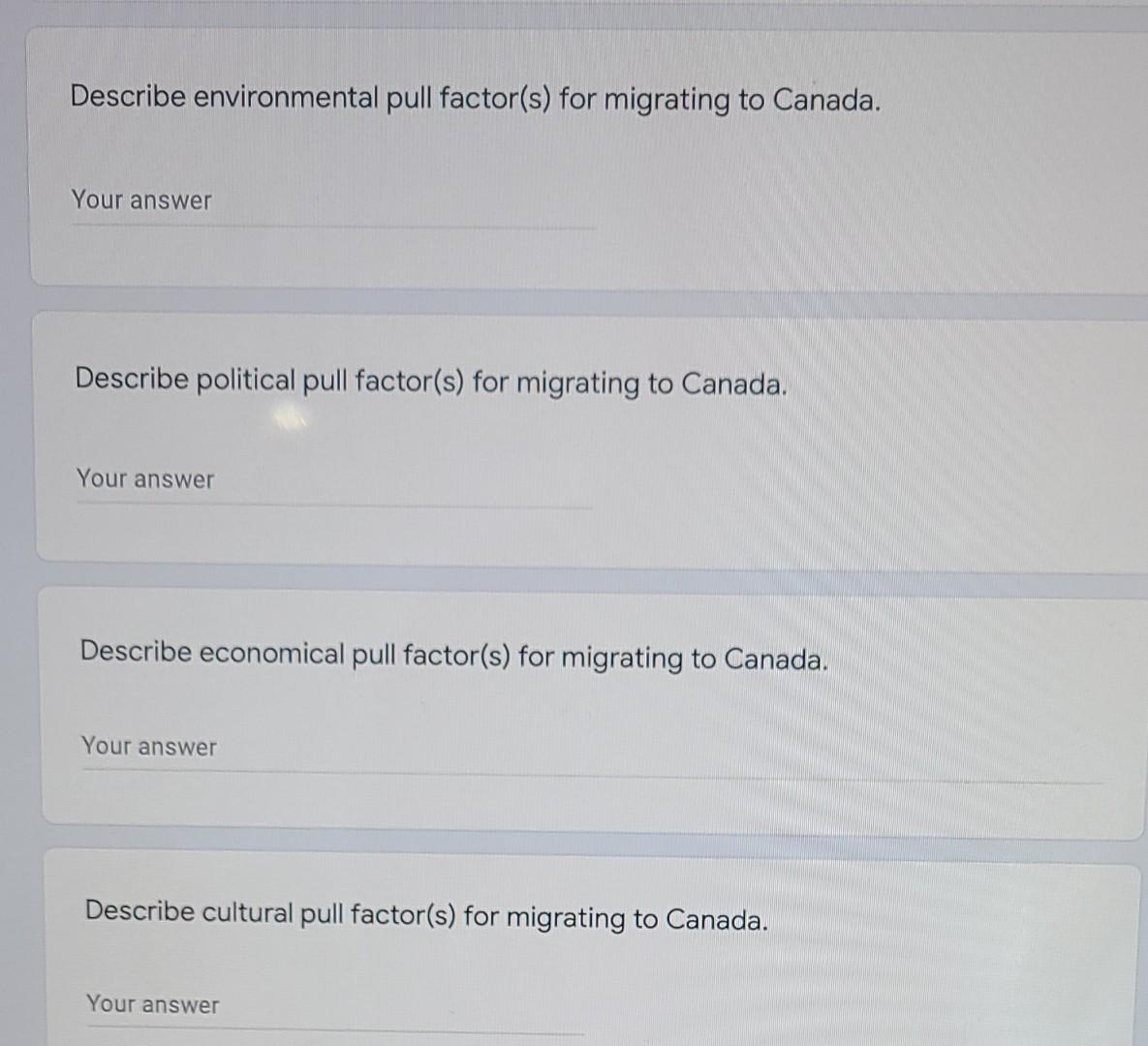The photo captures a computer screen, seemingly photographed using a phone. The screen background is a light gray color. Superimposed on this background are four vertically stacked rectangular boxes, each with rounded corners.

- **First Box**:
  - *Header Text*: "Describe environmental pull factor(s) for migrating to Canada."
  - *Subtext*: "Your answer."

- **Second Box**:
  - *Header Text*: "Describe political pull factor(s) for migrating to Canada."
  - *Subtext*: "Your answer."

- **Third Box**:
  - *Header Text*: "Describe economic pull factor(s) for migrating to Canada."
  - *Subtext*: "Your answer."

- **Fourth Box**:
  - *Header Text*: "Describe cultural pull factor(s) for migrating to Canada."
  - *Subtext*: "Your answer."

Each box has bold black header text in the upper half and a smaller, unbolded dark gray or black text below, over a light gray dividing line. The visible prompts in the boxes indicate that the image is likely part of a questionnaire or survey related to migration factors to Canada.